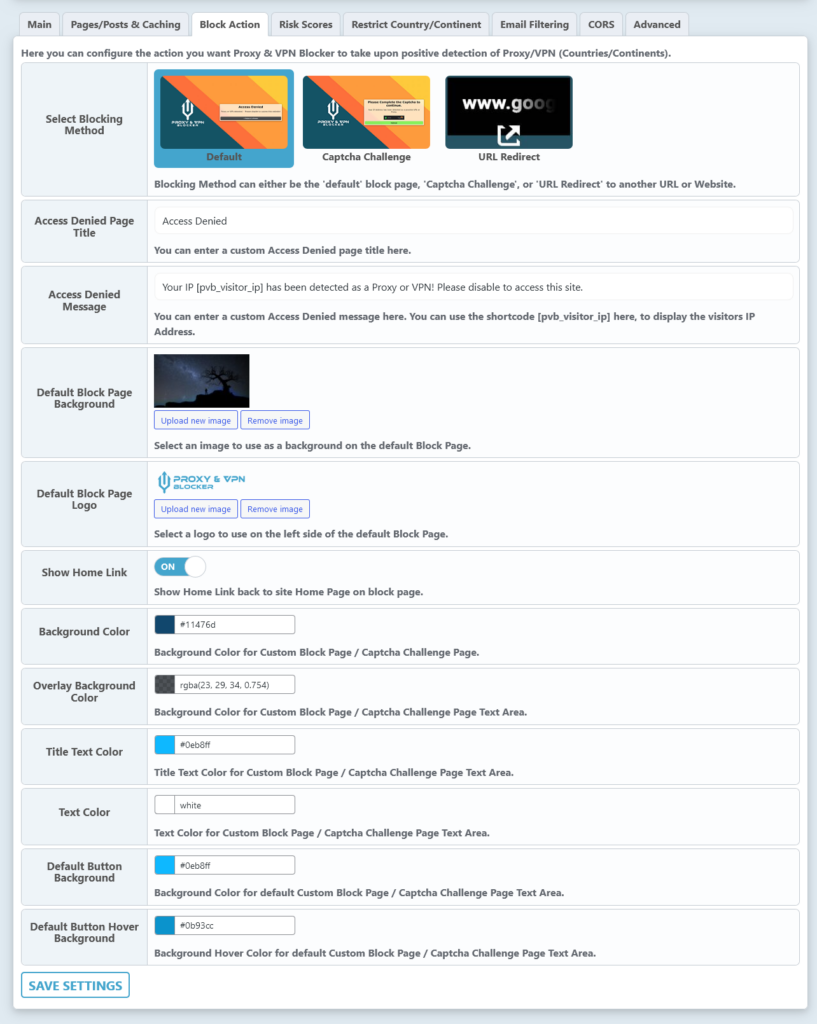**Detailed Caption for VPN Proxy Settings Page:**

The image displays a comprehensive VPN proxy settings page. At the top, there are several menu option tabs labeled: **Main**, **Pages and Post Caching**, **Block Caching**, **Risk Scores**, **Restrict Country/Continent**, **Email Filtering**, **CRS Cores**, and **Advanced**.

Below these tabs is the "Block Action Page" settings section, which includes various customizable options:

- **Select Blocking Method**: Options available are Default, CAPTCHA, Challenge, or URL Redirect.
- **Access Denied Page**: Here, you can enter a custom title for the access denied page.
- **Access Denied Message**: Option to input a custom message for the access denied page.
- **Default Block Page Background**: Image setting that displays a night sky with a person next to a dead tree.
- **Default Block Page Logo**: Set to display the "Voxie VPN Blocker" logo.
- **Show Home Link**: This option is switched on.
- **Background Color**: Set to #11476D (a specific shade of blue).
- **Overlay Background Color**: Set to black or RGBA(23, 29, 34, 0.754).
- **Title Text Color**: Set to #0EB8FF, a light blue color.
- **Text Color**: Set to white.
- **Default Message Background**: Set to #0EBDFF, another light blue shade.
- **Default Button Hover Color**: Set to #0B3C90, a dark blue shade.

At the bottom left of the settings panel is a small blue button labeled "Save Settings." This button is used to save any changes made to the settings.